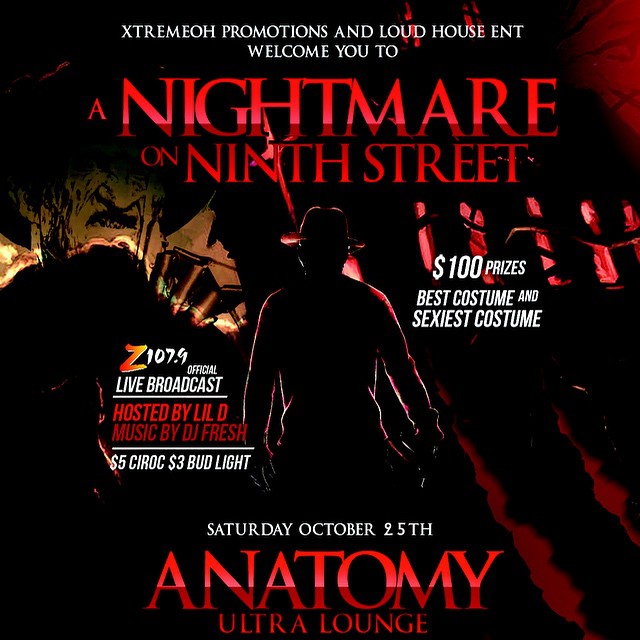The poster is a square image advertising a performance or event, most likely a Halloween-themed party. The background is predominantly dark with contrasting swaths of red and yellow resembling flames, creating an ominous atmosphere. At the top, in white text, it reads, "Extreme Promotions and Loud House ENT welcomes you to," and below this, in large, bold red letters, it states, "A Nightmare on Ninth Street," a clear homage to the horror film "A Nightmare on Elm Street." 

The centerpiece features a silhouette of a menacing figure in a fedora hat, reminiscent of Freddy Krueger, set against a haunting backdrop. Further down, in large red letters, the location is specified as "Anatomy Ultra Lounge." Above this, in white letters, the event date is displayed, suggesting it's a significant spooky celebration. 

Additional details in white text on the poster include mentions of $100 in prizes for best and sexiest costumes, with official broadcast by Z 107.9 hosted by Lil D and music from DJ Fresh. Drink specials are also highlighted, including $5 Crock and $3 Bud Lights. The overall design and text elements convey a chilling, Halloween party vibe.